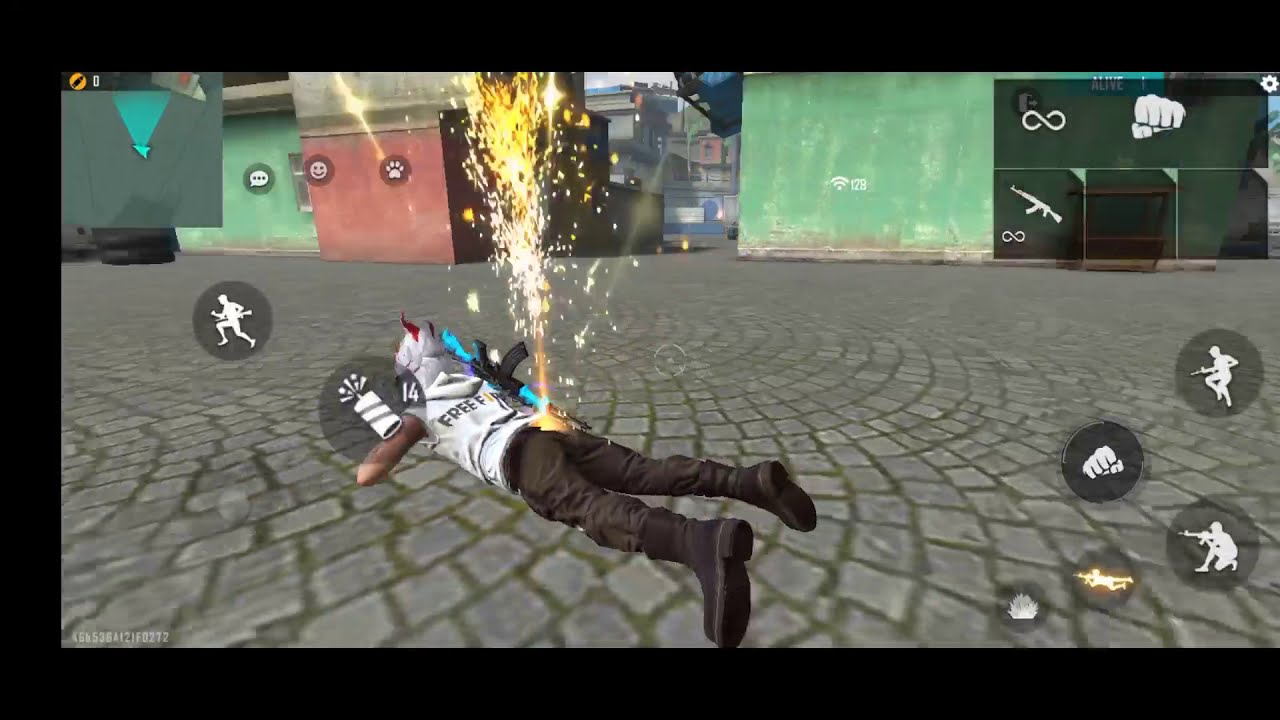In the image, a screenshot from a mobile video game, we see a character lying prone on a gray, paved walkway adorned with interlocking paving stones that form a spiral pattern. The character is dressed in black pants, black boots, and a white sleeveless hoodie with something written on the front, possibly "FREE." He also wears a distinctive hat, described as a small white hat with red spikes. A blue and black gun is strapped to his back.

Fire appears to be erupting from the character’s backside, creating a spray of yellow, sparkly flames that shoot upwards towards the sky. The background includes green and reddish-pink walls with some rectangular shapes near the top-left corner, along with various game interface elements. 

In the upper right corner, a menu icon is visible, along with several functional game icons scattered on the right and left sides of the screen. These include a fist, a gun, a firecracker, and a running figure, which suggests the different actions or abilities available to the player. The icon of a person crawling is highlighted in yellow, indicating the current action the character is performing.

Overall, the vivid depiction combines humor and chaos, illustrating a moment frozen in the midst of a dynamic and entertaining mobile gaming experience.